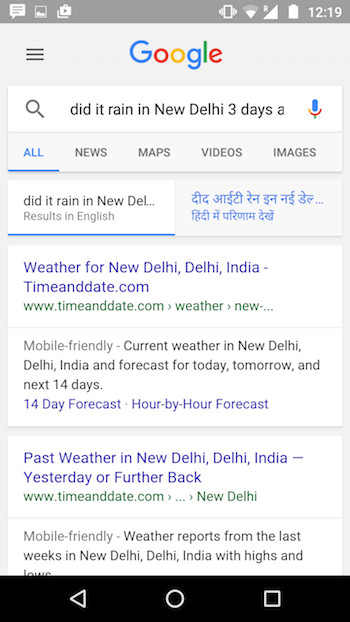Here is the cleaned-up and detailed caption for the image described:

---

A mobile screenshot of a Google search query is displayed on a white background. At the top of the screen, the Google logo is visible along with several lines of navigation. Below, the search bar prominently shows the query "Did it rain in New Delhi three days," truncated at the end with "A." To the left of the search bar icon is a magnifying glass, and to the right is a microphone symbol.

A line below the search bar separates it from the tabs labeled "All," "News," "Maps," "Videos," and "Images." Following this, another box mentions search results in English, with partial text indicating, "Did it rain in New Delhi?" and additional results in another language, likely Hindi, highlighted in blue.

Scrolling down, the first search result comes from timeanddate.com, offering detailed weather information for New Delhi, India. The snippet reads "Weather for New Delhi, Delhi, India," and features various sub-links like "Current Weather in New Delhi, Delhi, India," "14 days forecast," and "Hour by hour forecast." Another link points to historical weather data with "Past weather in New Delhi, Delhi, India, yesterday or further back."

The screenshot also indicates the current device time in the top-right corner, showing 12:19 PM.